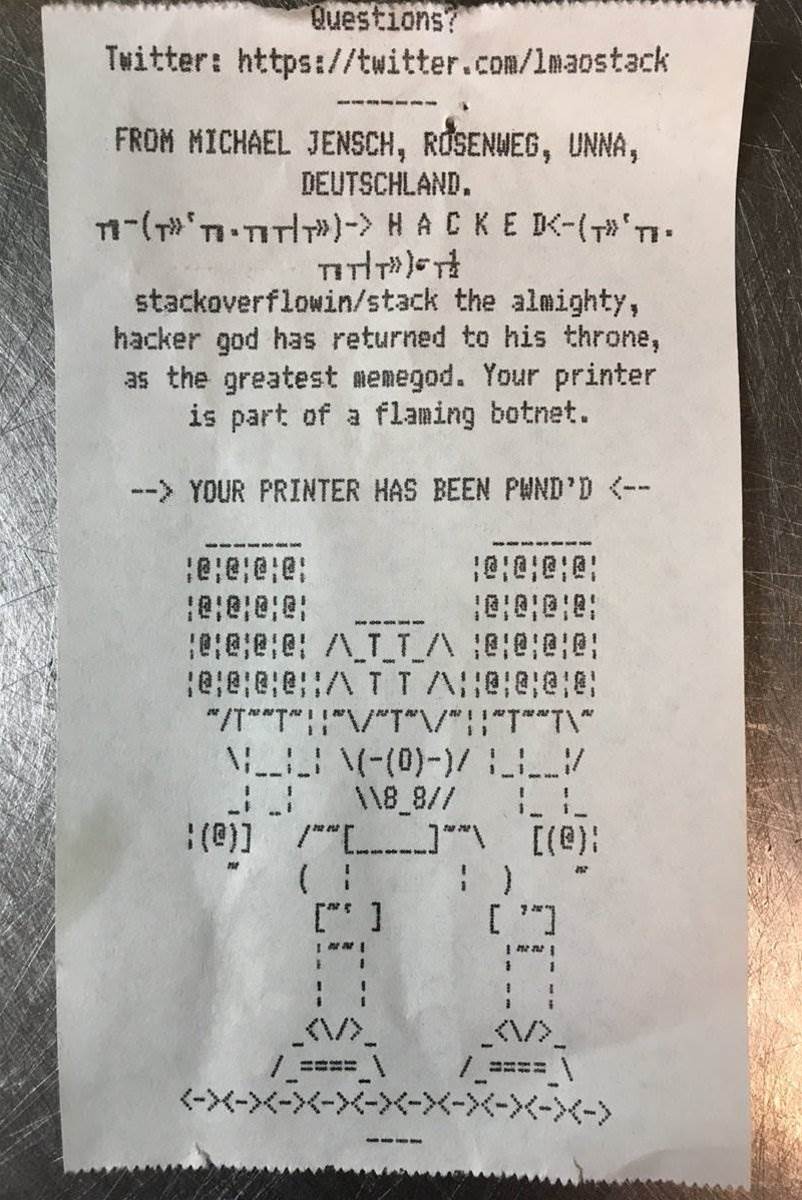This image shows a detailed receipt covered in printed text and symbols. At the top, it prominently displays the word "Questions?" followed by a URL: "Twitter: https://twitter.com/LMAOstack". Immediately below, it credits "From Michael Jentsch, Rosenweg Una, Deutschland". A series of symbols can be seen before the text "HACKED" in all caps. The message continues to read: "STACK OVERFLOWING/STACK THE ALMIGHTY, hacker god has returned to his throne, as the greatest meme god. Your printer is part of a flaming botnet." Midway through the receipt, arrows converge from all directions pointing towards the phrase "Your printer has been PWND'D" in capital letters. Further down, a pattern of symbols appears to form the shape of a robot with discernible legs and feet, adding a visual element to the text-heavy composition.